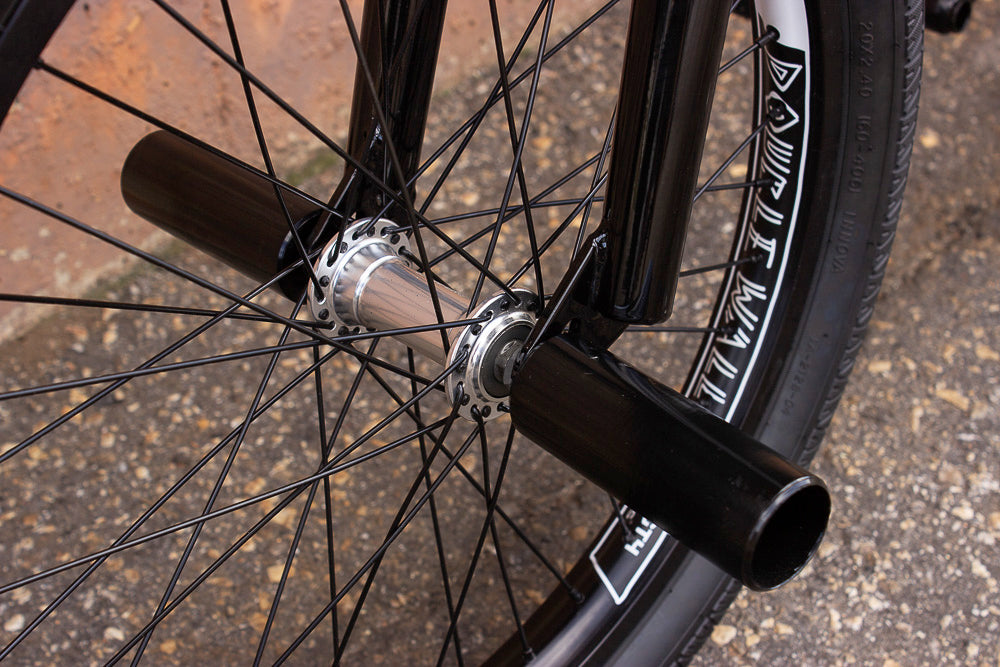This horizontally aligned rectangular close-up image features what appears to be the rear wheel of a bike, although there is some debate over whether it could be the front wheel due to the absence of gears and chain. The main focus is on the black, shiny cylindrical pegs that extend from the axle on both sides, typically used as footrests. You can see the black spokes radiating out from the wheel hub, with the tire itself appearing relatively new. The inner rim of the tire displays white geometrically-styled text that seems to say "Double Wall" and some additional, unreadable text. The bike is positioned on a speckled, rock-mixed sidewalk or graveled path. In the background, the image captures a portion of a black and gray asphalt street embedded with white and tan rocks, and a tan curb is visible in the upper left corner.